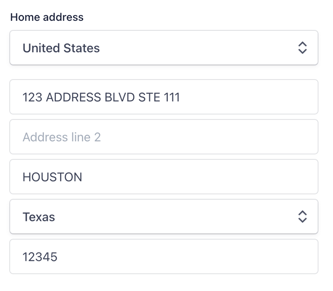A detailed image of a formatted address. The address reads:

"123 Address Boulevard, STE 111
Address Line 2
Houston, Texas 12345
United States"

The text is written in black and organized within outlined gray boxes. The boxes are placed on a white background. An arrow pointing up and down is featured next to "Texas."